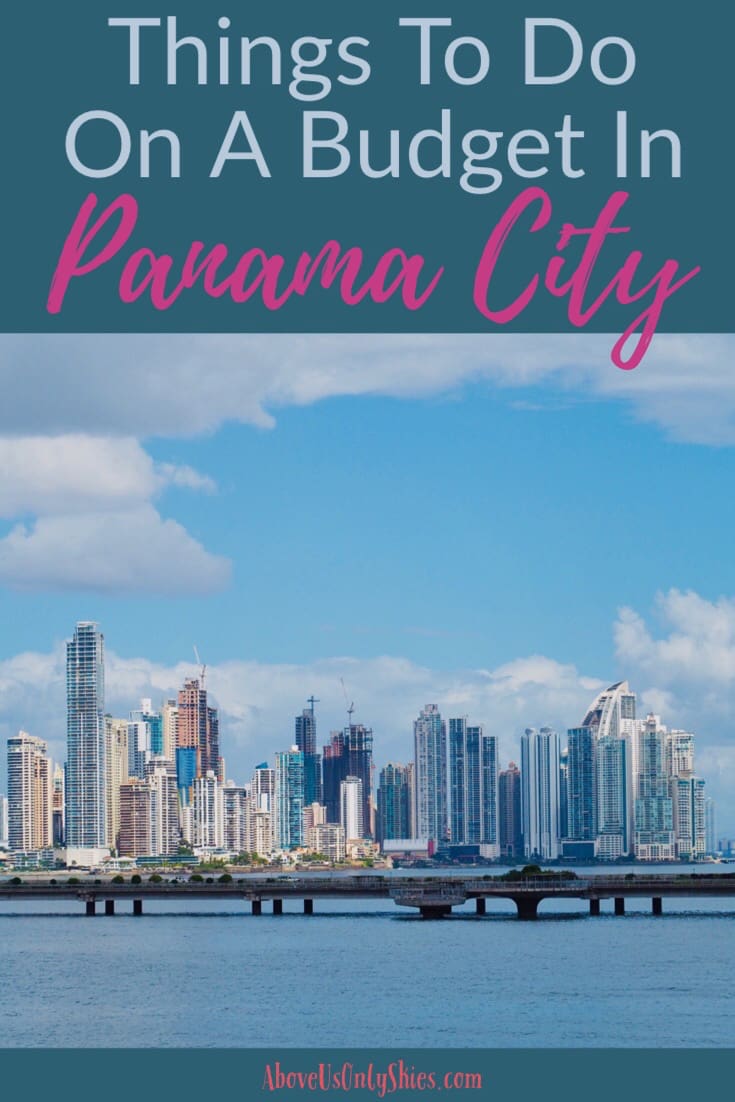The image features a top bluish-green rectangle containing the text "Things to Do on a Budget" in light blue. Below that, in pink cursive, "Panama City" is written, with the "Y" in "City" extending slightly below the rectangle. The central portion of the image depicts a panoramic view of a cityscape with numerous tall buildings in shades of silver, white, brown, cream, and blue. These skyscrapers are set against a backdrop of a blue sky dotted with puffy white clouds and some low-hanging clouds near the buildings. A long, dark bridge stretches across a body of water in the foreground, flanked by planters and trees. At the bottom, another bluish-green rectangle contains a cursive website name that is difficult to decipher.